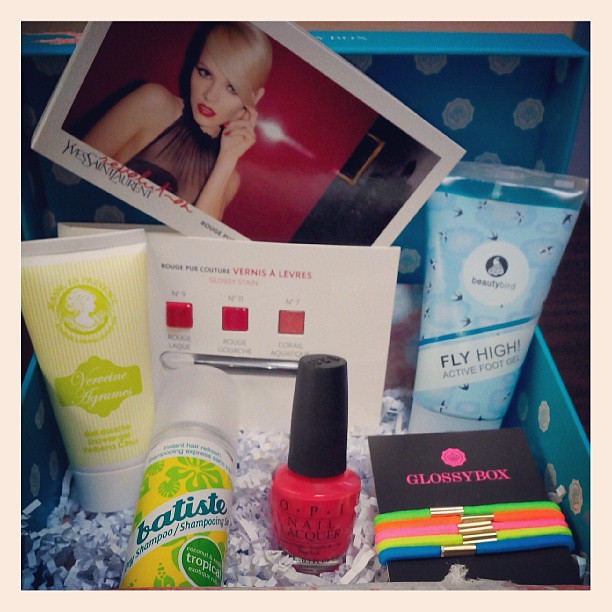The image depicts an opened beauty subscription box, primarily blue with a pattern of white, rose-shaped medallions. Inside, the box is lined with white shredded paper for cushioning. Featured prominently at the bottom right is a black piece of cardboard with "Glossy Box" written in pink text. Around this cardboard are various colored hair ties in light green, orange, pink, yellow, and blue. Among the products inside, there is a bottle labeled "Beauty Bird Fly High Active Foot Gel" and a dry shampoo from Batiste. Additionally, the box includes OPI Nail Lacquer and a small application brush, suggesting the presence of some nail care or cosmetics product. A stylish photograph of a model, wearing red lipstick and a sheer black dress against a red background, is included and marked with "Yves Saint Laurent." The box may also contain other beauty essentials like shampoo or body wash, evoking the essence of a curated beauty experience.